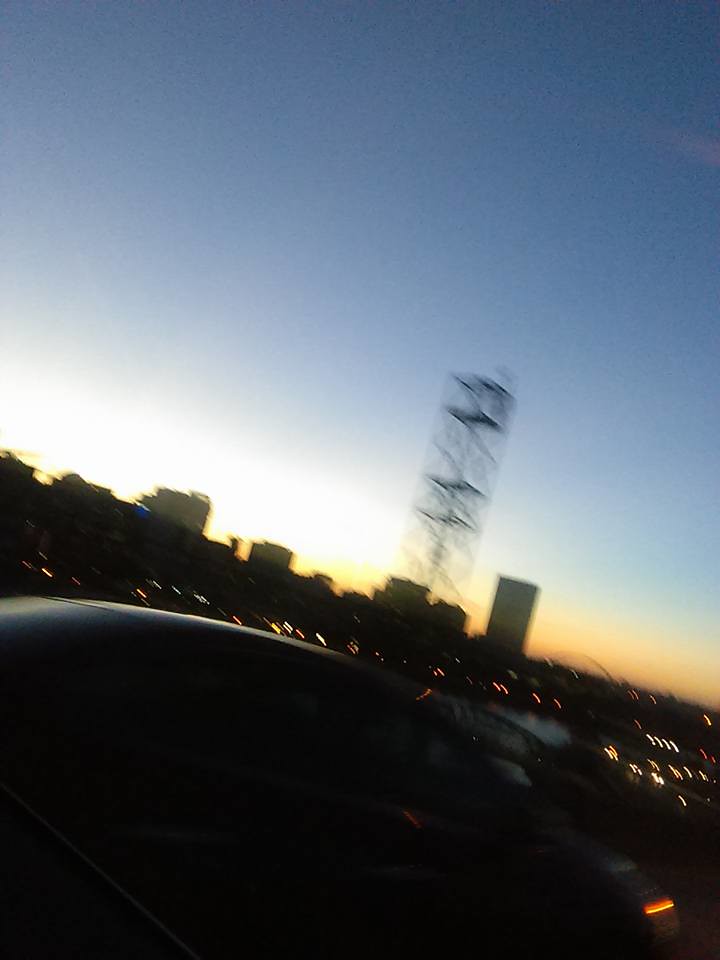The photograph captures a cityscape at dusk, taken from inside a dark-colored car with tinted windows, potentially while it was driving or parked in a lot. In the foreground, the car's side mirror is visible, giving context to the viewer’s vantage point. The image is blurry, suggesting motion or low light conditions as night falls. Below, you can see other vehicles on the road. Dominating the middle of the scene, there is a large, steel-framed structure resembling scaffolding or a trussed tower with visible stairs and various levels, though its exact purpose remains unclear due to the blur. The background showcases a city skyline with various high-rise buildings and a prominent, transparent steel tower, suggesting a mix of near-field and far-field elements. The tranquil blue sky transitions to an orange-yellow hue along the horizon, indicating the setting sun. Far in the distance, scattered lights begin to twinkle across the landscape, enhancing the city's evening vibe. A river or lake can be faintly made out beneath a trussed bridge, which connects the two shorelines far below.